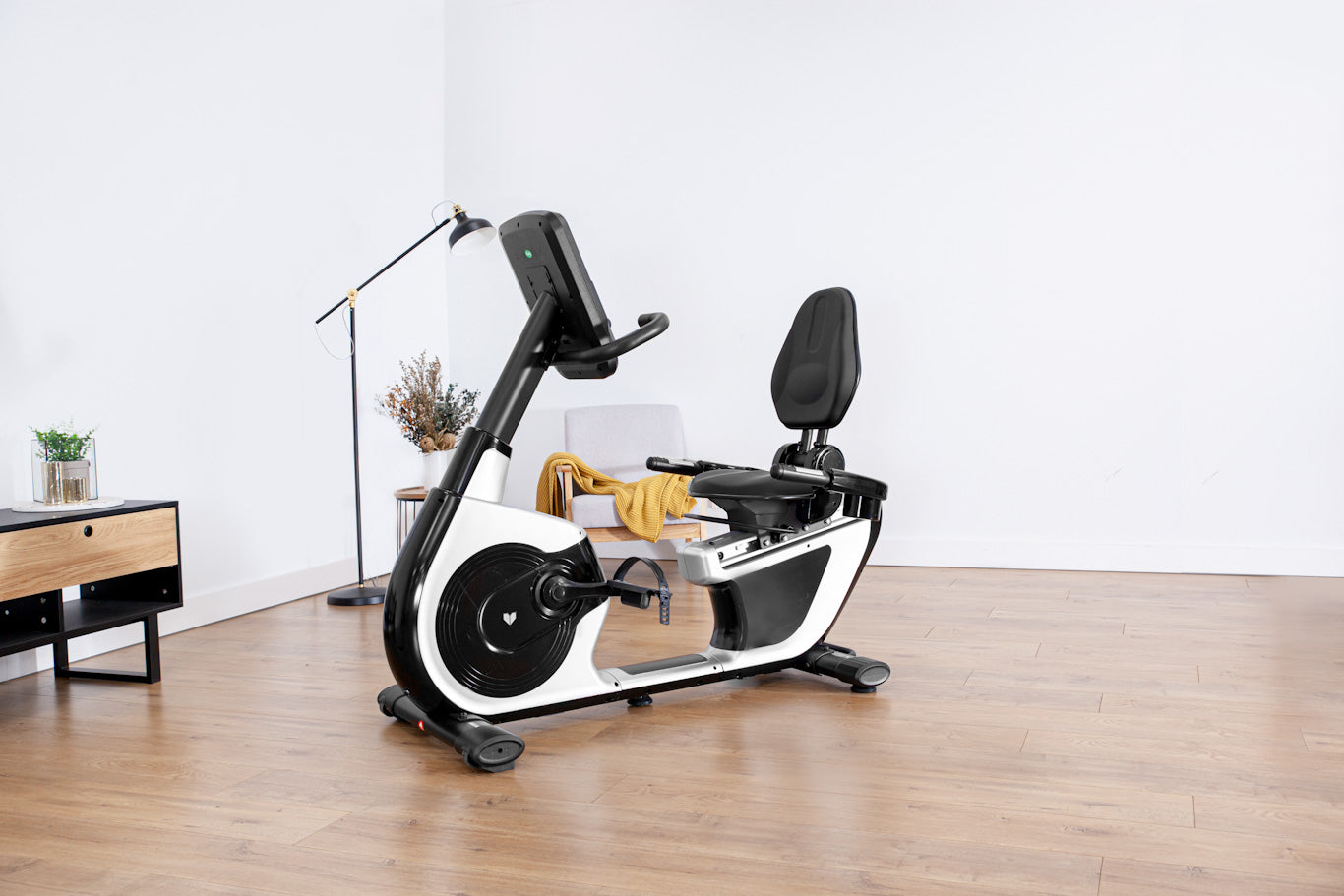The photograph captures a mostly empty room with clean, white walls and a light brown, wooden floor. In the center of the room is a black and white stationary exercise bike, equipped with a black seat and a control panel facing the user. The bike prominently features a towel draped over it, suggesting recent use. To the left of the bike, a black lamp stands tall next to a small table with a green plant. In the corner, a small gray chair adorned with a yellow blanket adds a cozy touch. Additionally, an end table adjacent to the wall features a black base and a light brown drawer handle. The room is spacious, uncluttered, and filled with natural light.